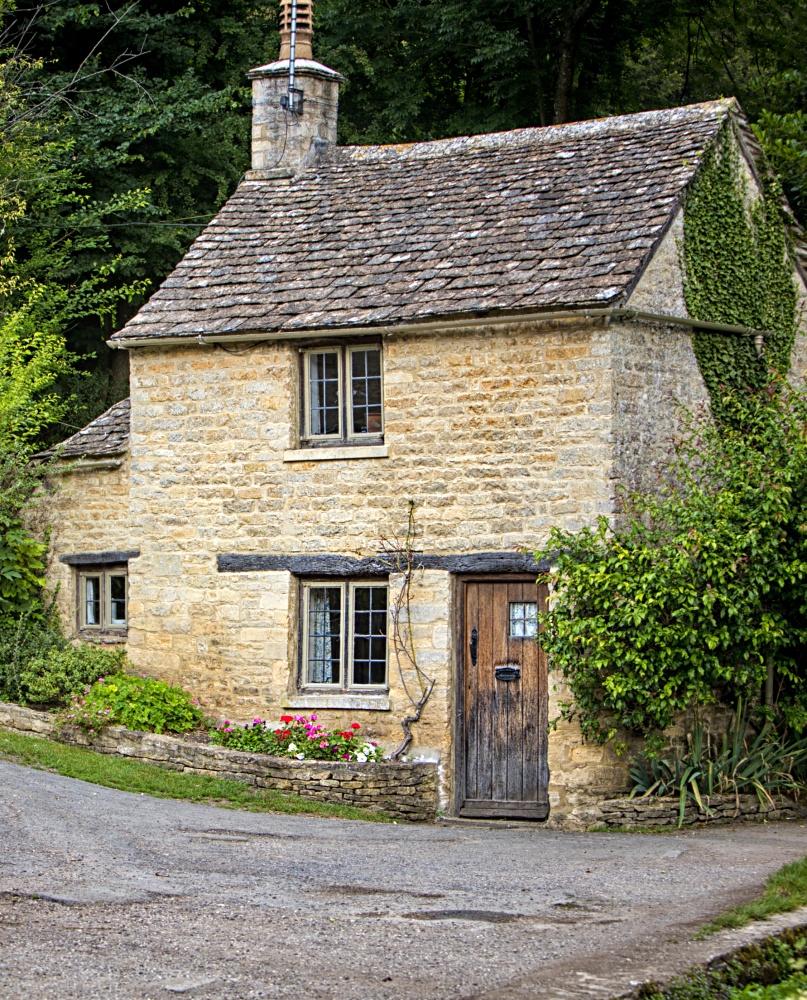This exterior photograph showcases a picturesque, quaint cottage reminiscent of old European, perhaps English, architecture. The main structure is a small, two-story square building constructed from brown stones, featuring a weathered brown wooden plank door with a small square window at the top right corner and an iron handle positioned slightly high on the left side. A mail slot is centered on the door. On the front facade, each story boasts a small window, one directly above the other.

To the lower right of the door, ivy and shrubbery climb the wall, while on the left, a charming raised flower bed constructed from a short rock wall burgeons with pink flowers, enhancing the cottage's rustic appeal. A diminutive one-story wing extends just beyond the left edge of the main building, contributing to the quaint charm with its own window.

The gray shingle roof, crowned by a chimney on the left end, adds to the cottage's historic look. The surrounding area features a curving driveway that nearly touches the front doorstep, bordered by lush, towering trees and vibrant greenery that envelop the scene in a serene, natural embrace.